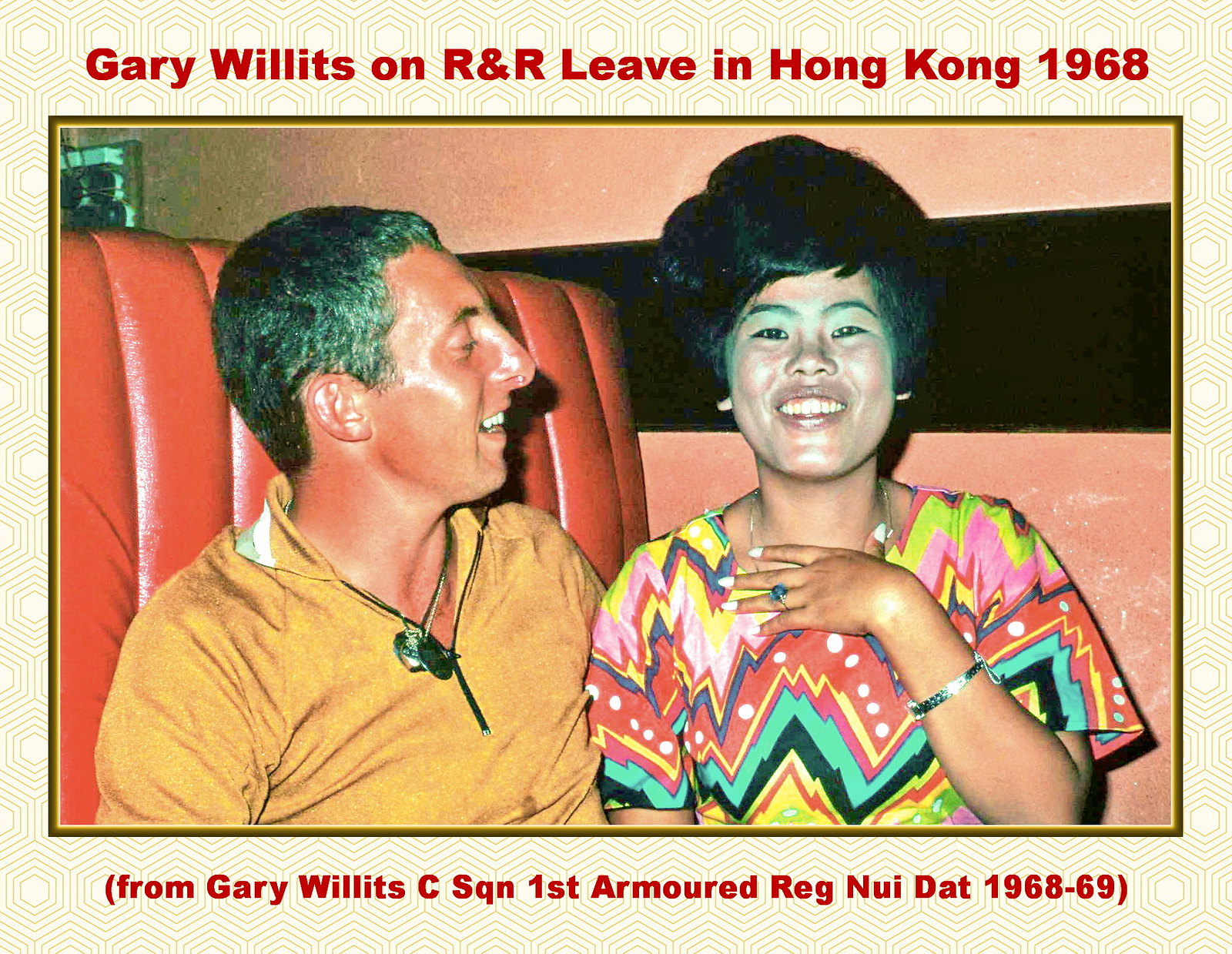The image depicts an indoor setting from 1968, showing a man and a woman seated at a booth in what looks like a diner or restaurant in Hong Kong. At the top of the image, a caption identifies the man as Gary Willits on R&R leave in Hong Kong, 1968, and a note at the bottom mentions "C SQN, First Armored Reg, Nui Dat, 1968-69." Gary, a Caucasian male, is sitting on the left, dressed in a mustard-yellow collared shirt with two necklaces, including dog tags, visible around his neck. He is smiling, and you can see his teeth as he looks towards the woman to his right. She is an attractive Asian female with dark hair styled in a 60s quaff, smiling warmly at the camera with her teeth visible. She rests her hand by her neck, showcasing white-painted fingernails and a silver bracelet. She wears a vibrant, colorful top featuring zigzags and dots in shades of red, yellow, turquoise, blue, black, and pink. The booth seat they share is upholstered in a red, leather-like material, contrasting with the pink wall behind them that is accented by a bold black stripe. The scene is a vivid representation of its time, capturing a joyful moment during Gary's leave.